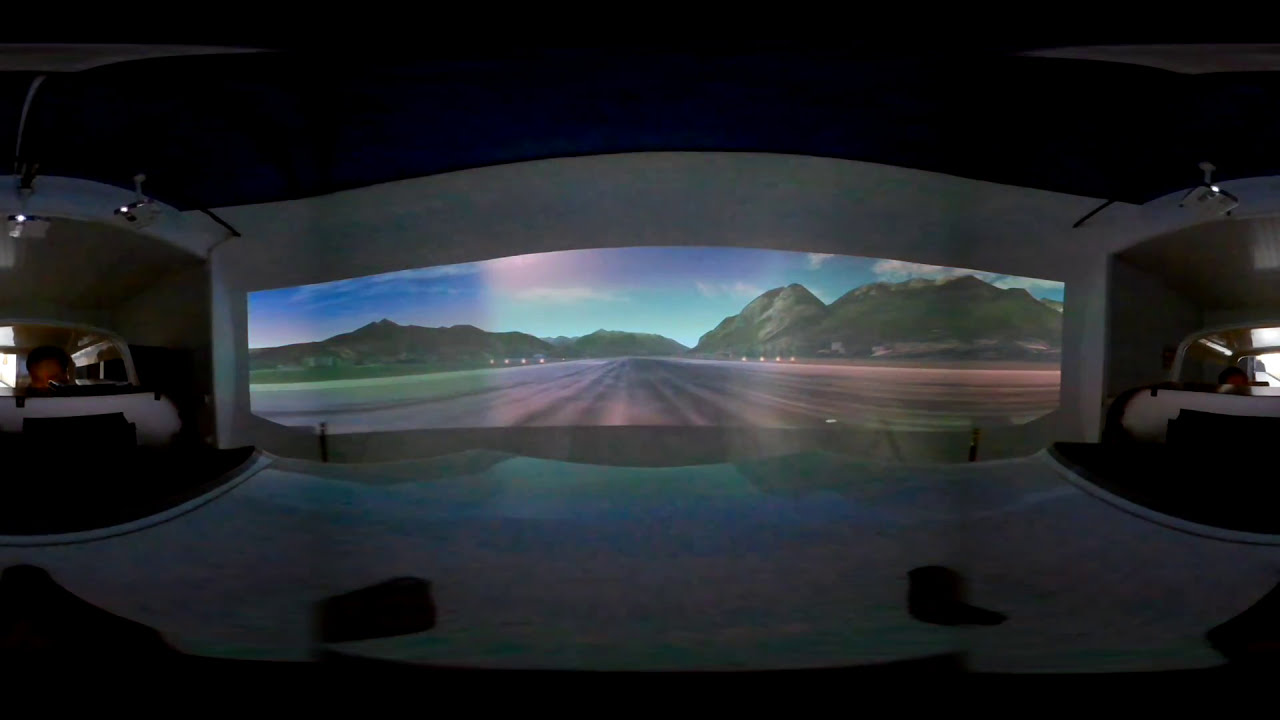The image depicts an indoor, dark room setup resembling a flight or driving simulator. At the center, a long and narrow horizontal image is projected onto a white wall, simulating a journey down an empty road or runway. This projection includes a detailed scene featuring a road flanked by four lights on each side, leading towards a distant mountain range under a bright blue sky with scattered white clouds. Below the projection, white fabric spreads on the ground, accompanied by various white machines and light fixtures hanging from a black ceiling. On the left and right sides of the room, there are toy-like cars or similar devices that appear to have screens showing the same projected scene. The atmosphere suggests a highly immersive experience, possibly for training or entertainment purposes. To the far left, there might be a person present, further adding to the realistic simulation setting.